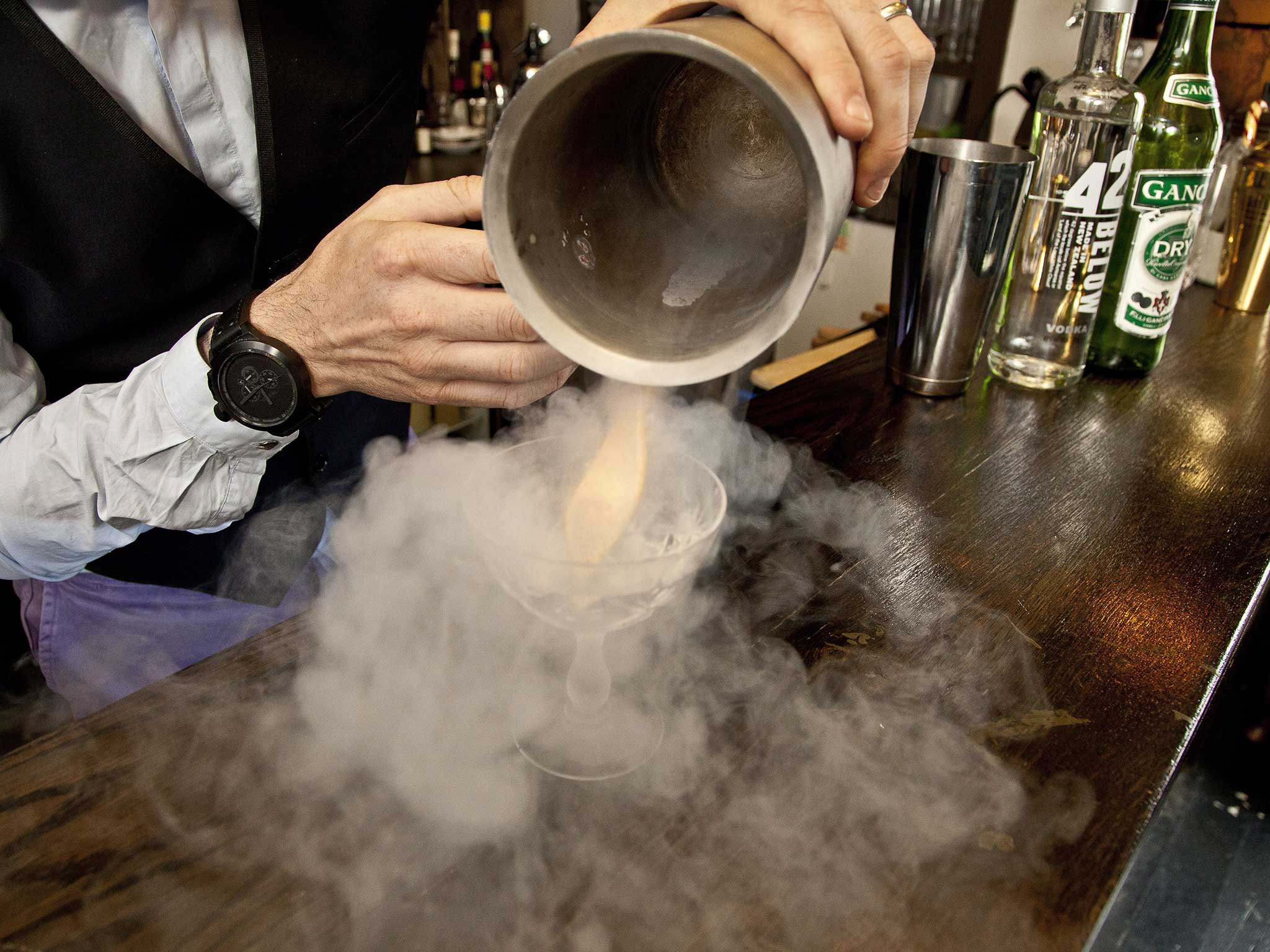In the image, a bartender is in the midst of pouring a drink from a large silver container into a small clear glass on a dark brown wooden bar top. The bartender, only visible from the chest down, is wearing a black vest over a light blue, possibly wrinkled, button-up shirt, combined with jeans and a large black watch on their wrist. The scene is dominated by the dramatic visual of thick white steam or smoke, likely from dry ice, billowing from the glass and enveloping the entire bar area. To the right of the bartender, the bar counter holds several items including a clear martini glass, another glass container, a bottle of vodka labeled "42 Below," and a green bottle of alcohol. In the background, there are additional alcohol bottles, contributing to the well-stocked and busy atmosphere of the bar. The bartender seems engaged in an intricate pouring process, adding to the theatrical ambiance created by the rolling mist of dry ice, which also forms frost on the container being used.